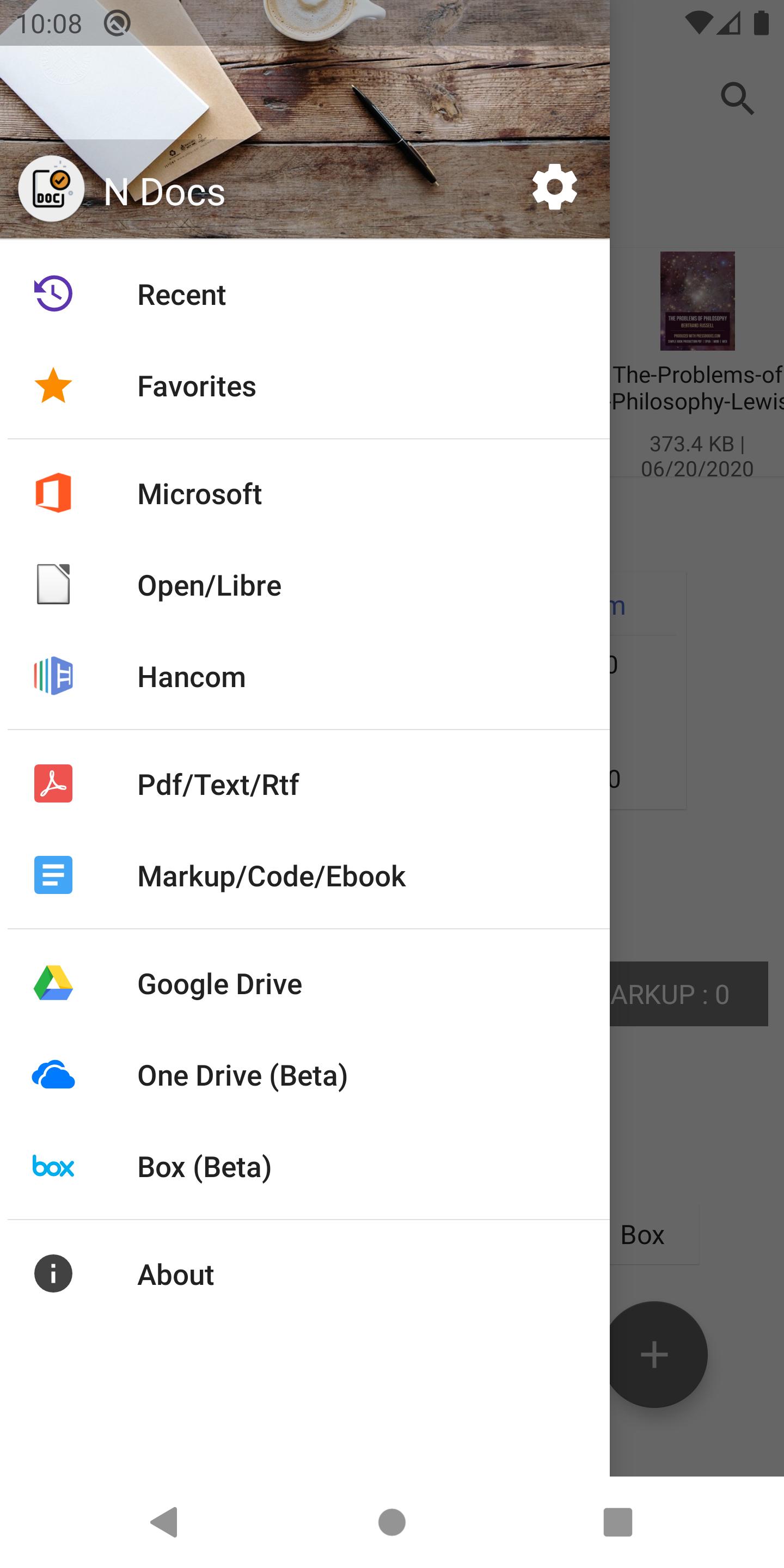Screenshot of the Endoc application interface displayed on a computer screen. The user interface features a wooden tabletop background with two notepads and a pen, creating a realistic workspace aesthetic. Prominently displayed is the "Endoc" logo. Beneath the logo, there are several navigational options or buttons, including "Recent," "Favorites," "Microsoft," "Oprah," "Libra," "Handcone," "PDF," "Text," "RTF," "Markup Code," "Ebook," "Google Drive," "OneDrive," "Box," and "About," each accompanied by their respective icons. The background shows a faint overlay, suggesting another page or window is open behind the main interface. Part of a search box and a thumbnail for a document titled "The Problems of Philosophy" by Lewis is barely visible along the right edge, hinting at multitasking or an opened document in the underlying window. The design primarily features a clean white background with black text, enhancing readability and focus on the app's functionalities.